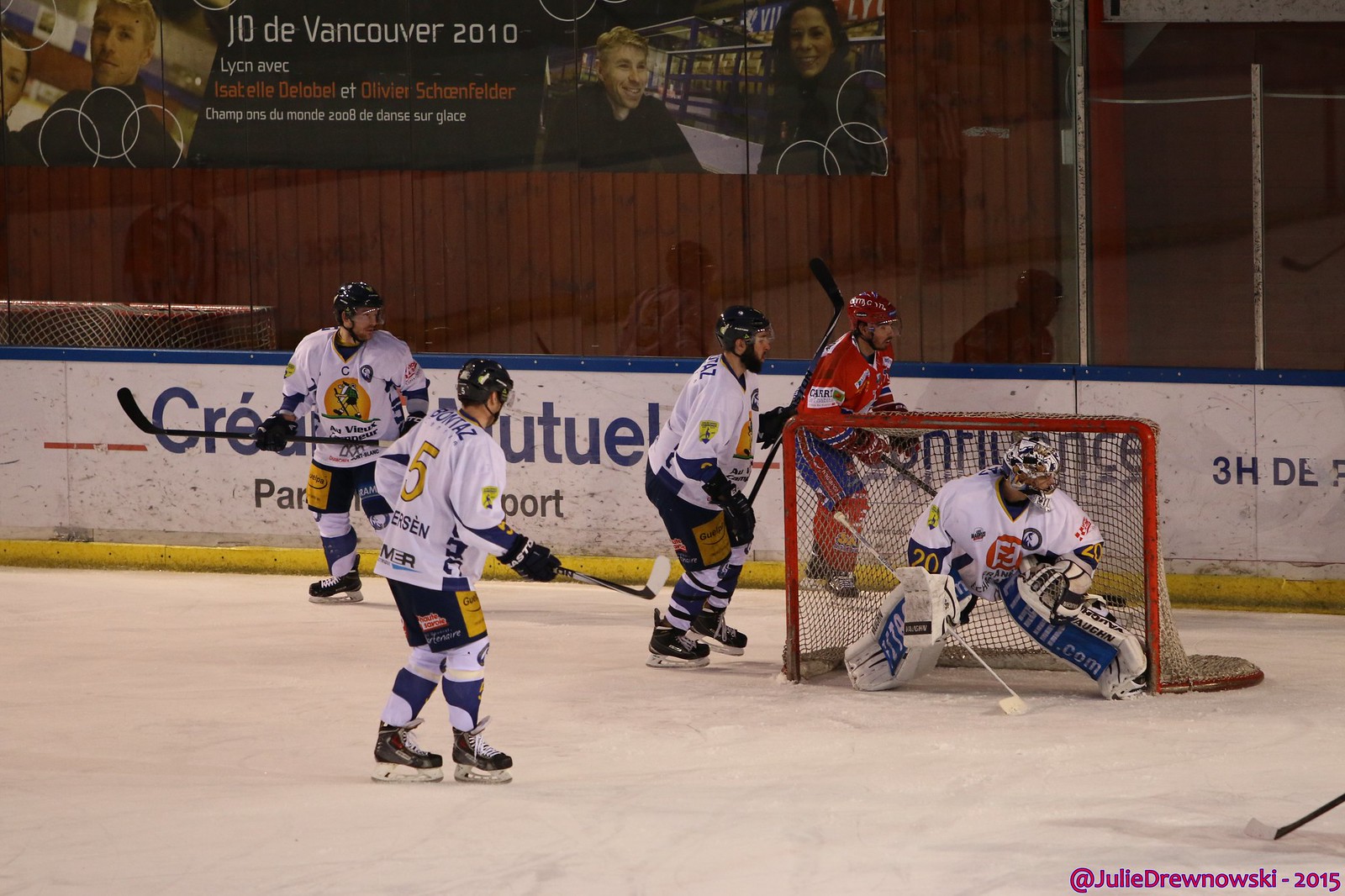This photograph captures an intense moment during an ice hockey game, presented in a horizontal-rectangular frame. In the middle of the action, four players from the same team, dressed in white jerseys and black shorts, are seen on the ice, all equipped with black helmets and skates. One of these players, distinguished as the goalie, is crouched in the goal with a larger stick poised for defense. Just behind the goal, an opposing player in a red jersey and royal blue shorts positions himself, ready to challenge the defense. The arena is detailed with clear plexiglass shielding, offering a glimpse of the scoreboard and spectators behind it. Above the rink, a prominent banner reads "J.O. Day Vancouver 2010," along with text in an unfamiliar language and images of a girl with dark hair and a blonde-headed boy. The perimeter of the ice features advertisements on a white wall, complementing the overall bustling ambiance of the game.